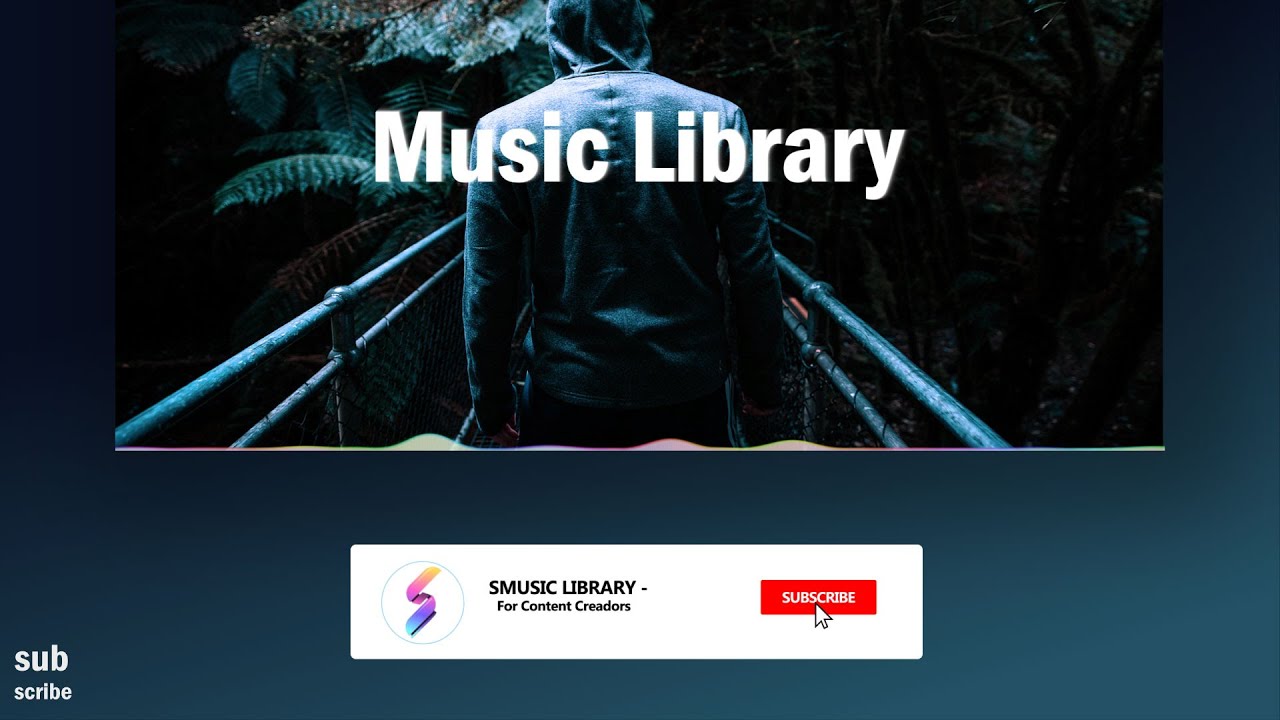The website features a striking image set against a dark, almost completely black background, with subtle touches of blue near the bottom. Dominating the scene is an enigmatic singer dressed in a dark sweatshirt with the hood up, partially obscuring his face. This singer is surrounded by lush, vibrant ferns, both in front and beside him, creating a stark contrast with the dark setting. 

The lighting is dramatic, with a single beam of light illuminating the singer from above, emphasizing his presence and casting intriguing shadows. The scene evokes a vintage maritime atmosphere, reminiscent of the Titanic, complete with old-fashioned railings on either side of him. The composition focuses on his upper body, as his legs are not visible, giving the impression that he might be leaning or sitting.

Prominently displayed behind him, in bold white letters outlined at shoulder level, are the words "Music Library." Below this, a colorful array of waves in pink, green, and yellow adds a splash of vibrancy to the otherwise dark image. Additionally, there's a white box with the text "S Music Library for Content Creators" inside it. Within this box, a circular element containing a multi-colored design comprising blue, pink, and yellow adds more visual interest.

An orange subscribe button, accompanied by an arrow pointing towards it, is notably visible, urging viewers to take action. In the lower right-hand corner, the word "SUBSCRIBE" is displayed, split across two lines, with "S-U-B" on one line and "SCRIBE" on the next. This meticulously designed image serves as a comprehensive visual invitation to explore the music library for content creators.